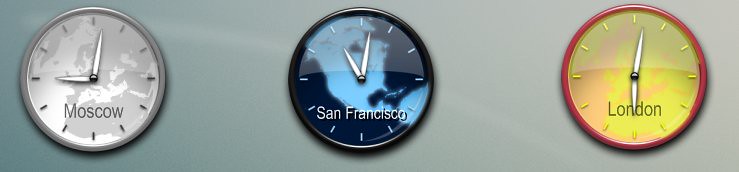The image is a wide, rectangular photograph displaying three equally spaced analog clocks against a smooth wall that transitions from mint green to a lighter shade towards the right. Each clock denotes a different time zone: Moscow, San Francisco, and London.

The Moscow clock on the left features a predominantly gray face with silver accents and hands, framed by a silver rim. Its face displays an outline of Russia and nearby continents. The clock shows two minutes past nine.

The center clock for San Francisco has a blue-themed face with a black rim. It includes an outline of North America, parts of Canada, South America, and Mexico, with variations of light and dark blue. This clock indicates the time as two minutes past eleven.

The London clock on the right has a vibrant face with a mix of orange, yellow, and pink hues, resembling a tie-dye or cloud-like effect. It is framed by a red rim and has silver hands. The clock shows six minutes past two.

Each clock lacks numerical markings, relying instead on lines to denote the hours, ensuring a sleek and modern design.